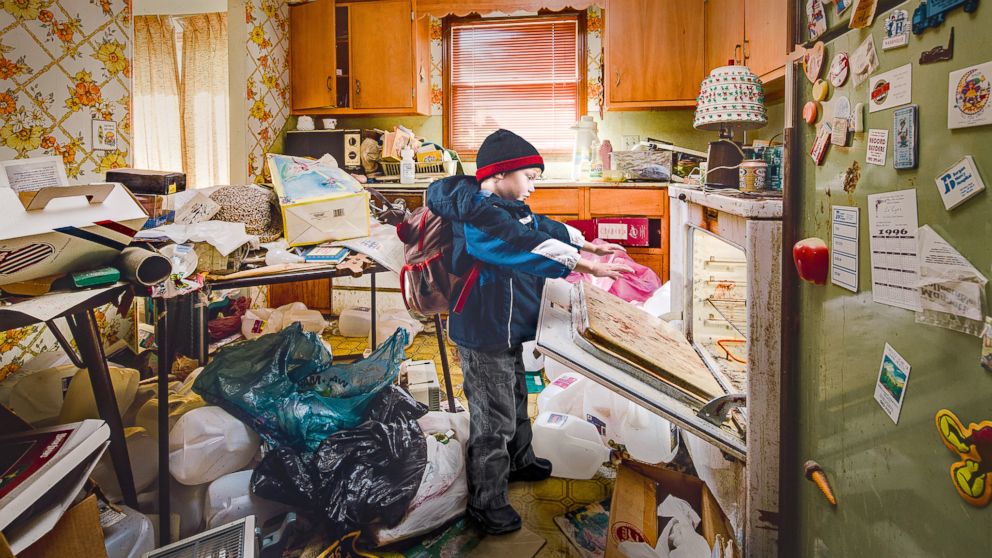In a cluttered, chaotic kitchen that resembles a scene from the show "Hoarders," a young boy in winter attire stands in front of an open, grime-covered oven, holding his hands out as if to warm himself. The space is overwhelmingly messy, with every surface and inch of floor covered in garbage, old food containers, and various household items. The boy wears a two-toned blue parka, a black beanie with a red stripe, a brown backpack with red trim, distressed black jeans, and winter boots. 

In the background, a metallic, magnet-covered refrigerator sits amidst the mess, along with a table heaped with trash, a black microwave, and wood cabinetry that is slightly ajar. The floor is a 1970s-style yellow squared linoleum, and the walls feature a grid patterned wallpaper adorned with orange and yellow flowers. The overall scene is one of severe disarray and neglect, capturing a moment of apparent need as the child tries to extract warmth from the oven amid the disorder.